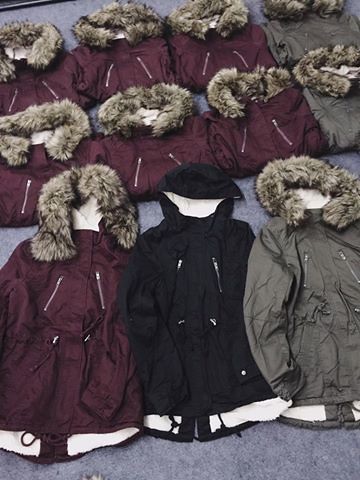This promotional image showcases a selection of winter parka jackets arranged in three distinct rows on a gray carpet. The foreground features three fully laid-out jackets in maroon, black, and gray, with the maroon and gray ones sporting fur-lined hoods, while the black one has a simple white lining. Each jacket is detailed with diagonal zippers on both sides of the chest and hips. The background displays two rows of folded jackets: six maroon parkas with fur hoods and two gray parkas positioned to the right. Overall, there are 11 jackets in the image, combining functionality with stylish appeal.